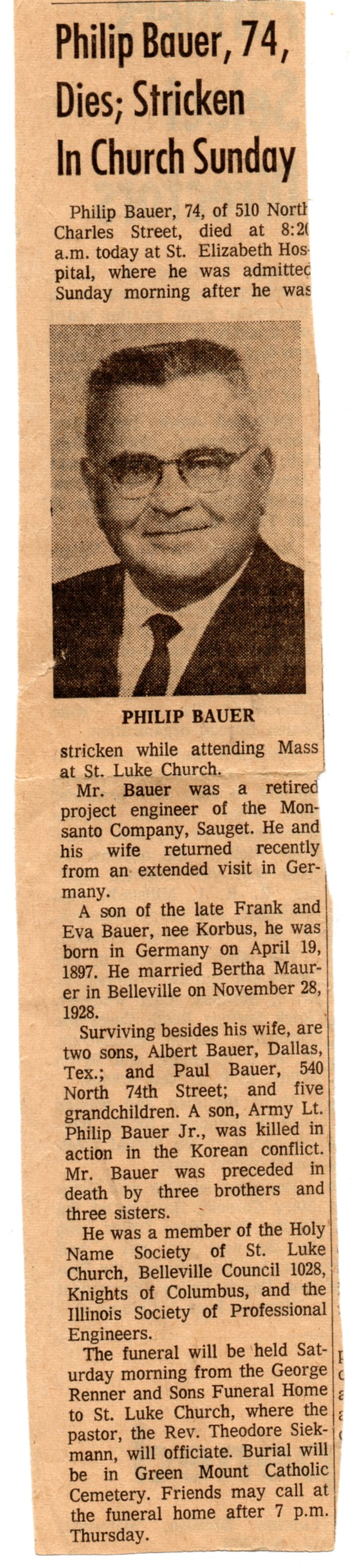The image is a scan of an aged, tannish-yellow newspaper clipping, specifically an obituary. The article's headline reads, "Philip Bauer, 74, dies stricken in church Sunday," followed by detailed black text. The obituary details that Philip Bauer, 74, of 510 North Charles Street, passed away at St. Elizabeth Hospital at 8:20 a.m. after being stricken while attending Mass at St. Luke Church. Philip Bauer, a retired project engineer from Monsanto Company in Sauget, had recently returned from an extended visit to Germany with his wife. The article also states that he was born in Germany on April 19, 1897, married Bertha Mauer in Belleville on November 28, 1928, and was preceded in death by a son, Army Lt. Philip Bauer Jr., killed in the Korean conflict, three brothers, and three sisters. He is survived by his wife, two sons—Albert Bauer from Dallas, Texas, and Robert Bauer from 540 North 74th Street—and five grandchildren. Philip Bauer was a member of the Holy Name Society of St. Luke Church, Belleville Council 1028 Knights of Columbus, and the Illinois Society of Professional Engineers. The funeral service was scheduled to be held on a Saturday morning, officiated by Rev. Theodore Seekhman at St. Luke Church, with burial at Green Mount Catholic Cemetery. Visitation was to start after 7 p.m. Thursday at George Renner and Son's Funeral Home. Additionally, the clipping includes a black-and-white portrait of Philip Bauer at the top, showcasing a well-built, elderly man with glasses, wearing a black suit, black tie, and white shirt, and sporting a neat crew cut.